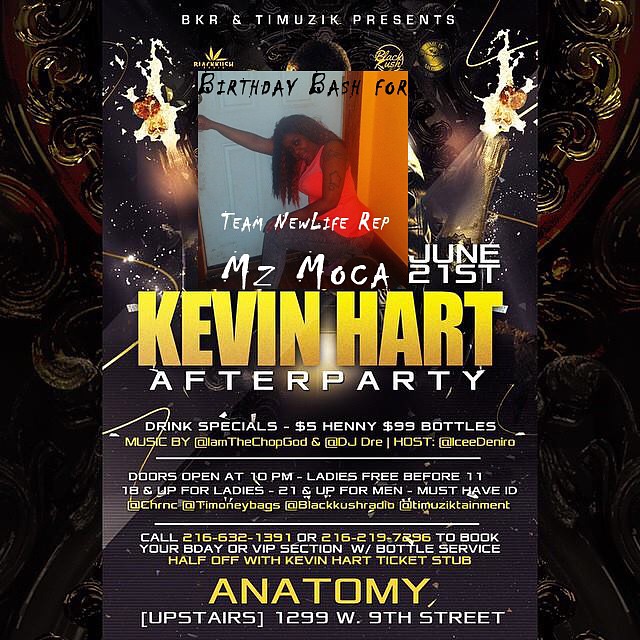The poster, advertising a bar event, features a dark, swirling background of gold and brown hues. Dominating the center is a vertical rectangular image with multiple pieces of relevant information. 

At the top, the text reads "BKR and Timusic Presents", followed by "Birthday Bash 4" in bold black letters. Just below that, it states "Team New Life Rep Ms. Mocha" in white. Positioned to the right, the date "June 21st" is also in white text.

Central to the poster is a picture of an African-American woman, identified as MZ Mocha. She is sitting down, with long hair, wearing an orange top and jeans, her right arm stretched in front of her, posing against an orange wall with a white door behind her.

Below this, in large yellow capital letters, it announces "KEVIN HART". Underneath, in white letters, it states "After Party". Further down, it lists detailed event information including drink specials like "$5.00 Hennessy and $99.00 bottles". It also mentions music by "I Am The Chop God and DJ Dre" and hosted by "I'll See DeNira". Additional details include "doors open at 10 p.m.", "ladies free before 11", "18 and up for ladies, 21 and up for men, must have ID". A call-to-action note highlights "call 216-632-1391 or 216-219-7296 to book your B-Day or VIP section with bottle service half off with Kevin Hart ticket stub".

At the very bottom, "ANATOMY" is displayed in large yellow capitals, followed by the location "upstairs 1299 West 9th Street" in smaller white text.